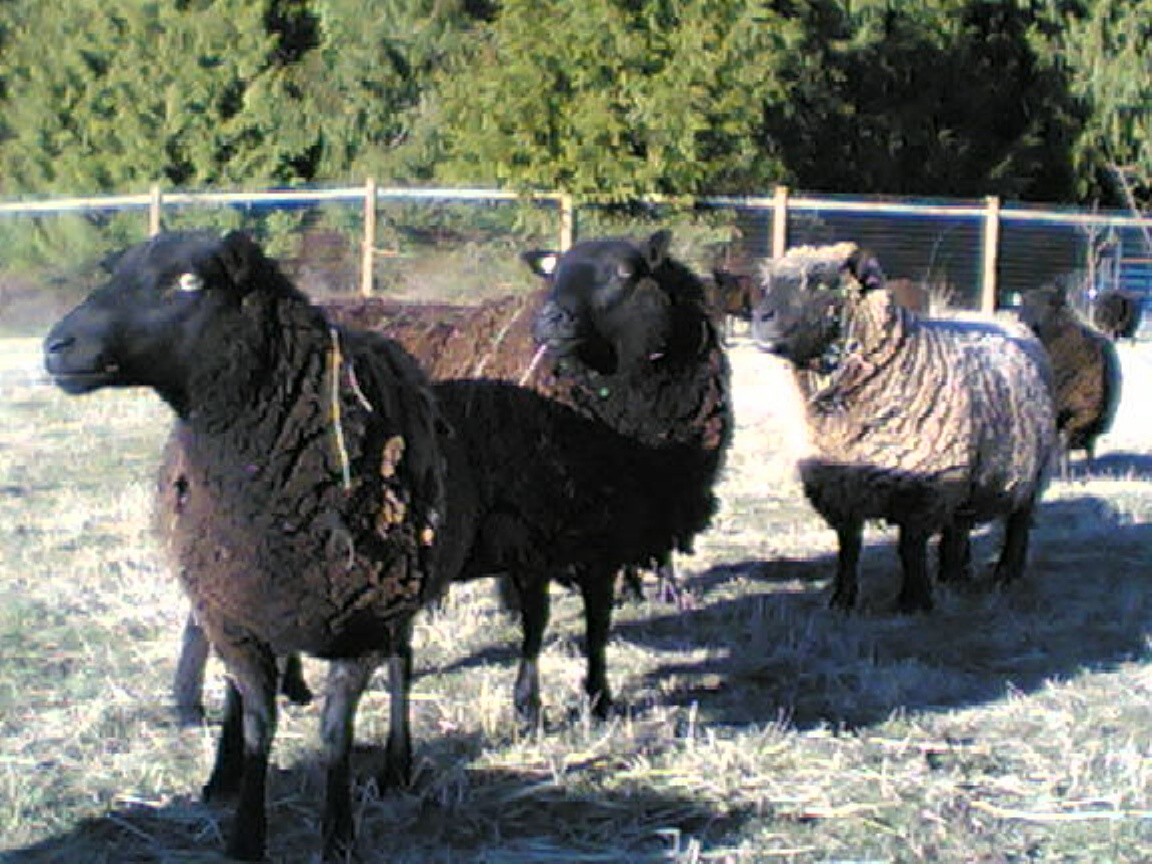This low-resolution photograph captures a peaceful pastoral scene featuring a grassy field enclosed by a wood-framed fence with wire interior fencing. The field's grass appears mostly dried and is interspersed with white hay, creating a speckled effect. Dominating the image are three sheep, framed against a backdrop of lush green trees. To the left, two black sheep stand close together; one faces the left with its head turned slightly towards the camera, revealing a prominent white eye and fluffy, black shaggy wool with bits of grass stuck to it. Slightly to their right stands another sheep, distinguished by its white wool, black face, and black legs, appearing brown and white mingled along its front. In the distance, there is another black sheep, slightly out of focus and looking away from the camera, near the top left of the image. The background is filled with tall, evergreen-style trees that tower over the scene, completing this picturesque country image.